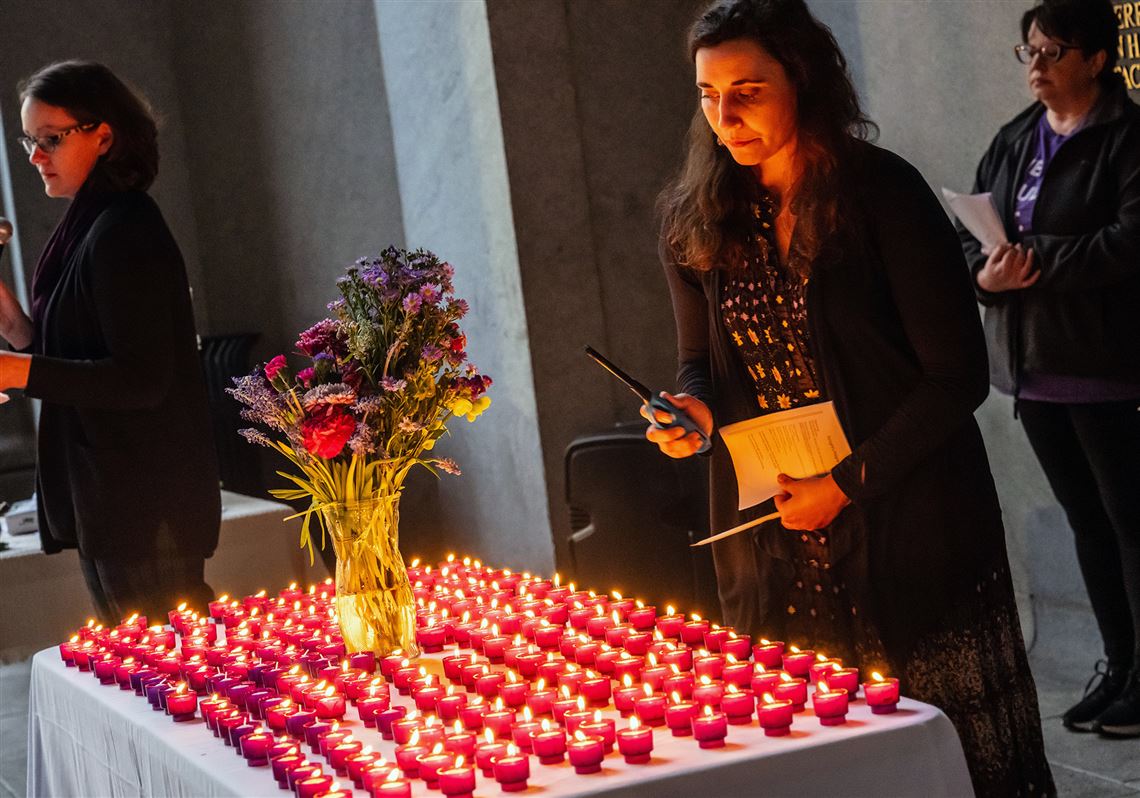In this poignant photograph, a central figure, a woman with long black hair dressed in a floral dress and a black cardigan, stands solemnly before a long table draped with a white tablecloth. The table is adorned with approximately 50 small red candles, all of them alight, casting a warm glow. Interspersed among the candles, there's a vase bursting with vibrant flowers in shades of red, pink, purple, and yellow. The woman in the foreground holds a barbecue-style lighter with an extended nose in her right hand, and a paper program, possibly related to the ceremony, in her left. To her right and slightly behind, another woman dressed in black, with short brown hair and glasses, stands against a wall, hands clasped around a similar program. Further to the left, a third woman faces sideways, contributing to the atmosphere of this solemn gathering. All participants are dressed in somber black attire, suggesting that the scene might be part of a funeral service, religious ceremony, or vigil.